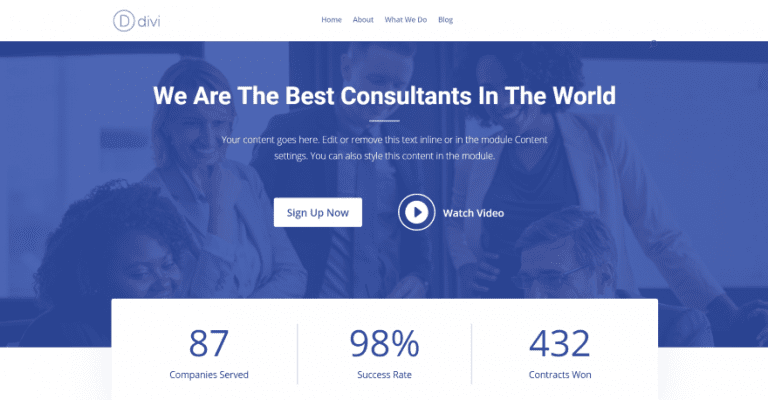The webpage seems to be a template for a website called "Divi." At the top, there is a large, circular logo featuring a capital 'D' in dark violet-purple. Next to this logo, the name "Divi" is written in lowercase letters. Centered on the page are navigation options for "Home," "About," "What We Do," and "Blog."

Dominating the center of the page is a large purple banner. The banner includes an image of several people gathered around a computer, all smiling and appearing engaged with whatever is on the screen. Overlaid on this image in bold white text are the words, "We are the best consultants in the world." Beneath this bold claim, there's placeholder text that reads, "Your content goes here. Edit or remove this text inline or in the module content settings. You can also style this content in the module."

Below the banner, a white button labeled "Sign Up Now" invites users to take action, while a play button labeled "Watch Video" suggests the presence of multimedia content. Under these buttons is a horizontal rectangular banner displaying statistics in the same dark violet-purple text: "87 companies served, 98% success rate, 432 contracts won."

From the provided details, it appears that this webpage is currently a work in progress. The placeholder text suggests that this template is customizable, allowing users to input their own content, indicating that it might be in the development or template stage, ready for someone to personalize and publish.